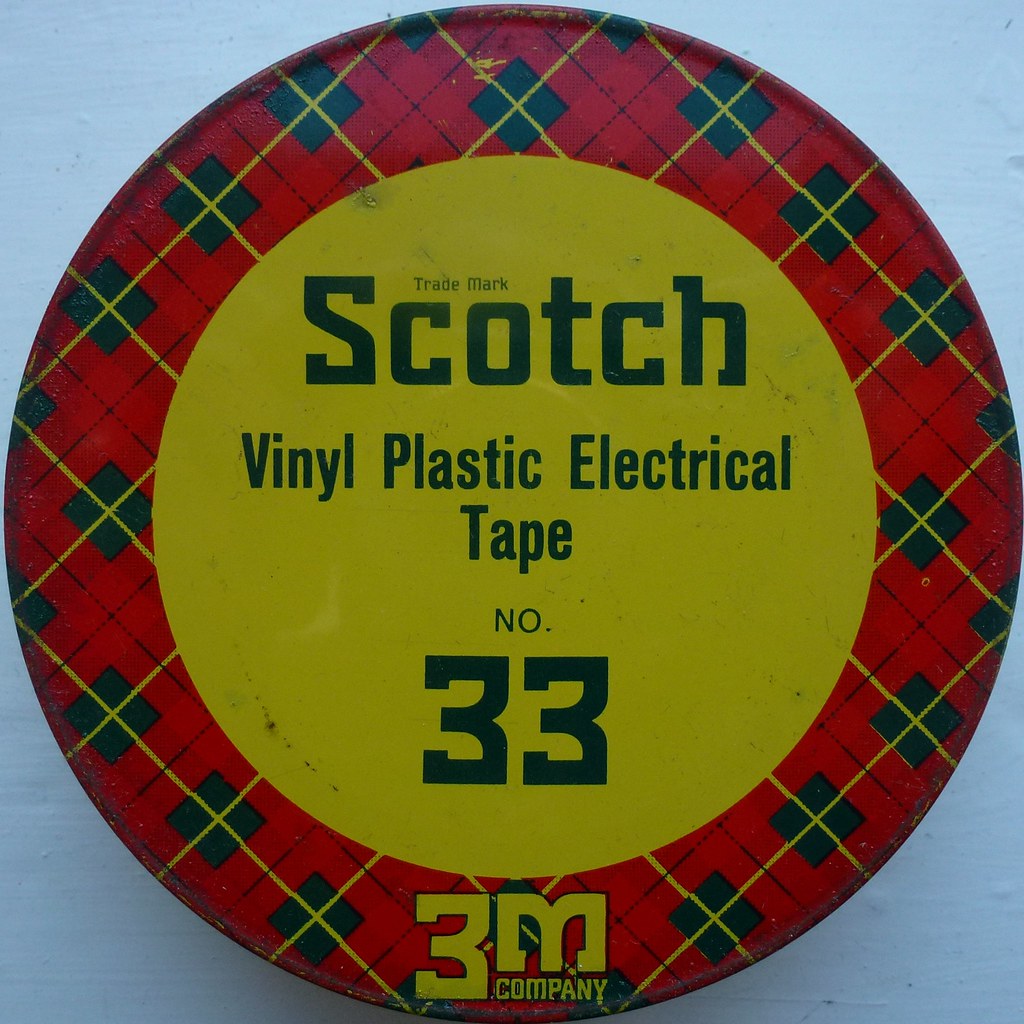This photograph showcases a vintage, unopened pack of Scotch Vinyl Plastic Electrical Tape number 33, resting on a probably wooden table painted white. The packaging is indicative of its age, likely several decades old, with visible signs of wear and damage. The design features a prominent yellow circle at the center, displaying the text "Scotch Vinyl Plastic Electrical Tape Number 33" in bold black letters. Below this, in smaller black text on the yellow circle, is the "3M Company" logo. Surrounding the central yellow circle is a vibrant, eye-catching pattern consisting of red, yellow, and green lines, along with black squares, creating a tartan plaid border. The overall style of the image is a color photograph with a focus on product packaging realism, emphasizing the intricate design details and vintage aesthetic of the tape's packaging.